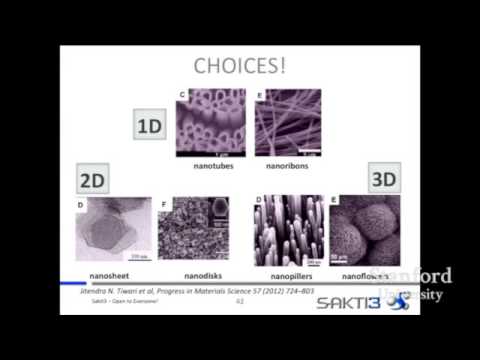The image is a PowerPoint slide with a white inner background bordered by a black frame. The title at the top reads "Choices!" in gray text. Below the title, there are six distinct microscopic images organized in two rows. The top row features two images under the label "1D" within a gray box. The first image shows nanotubes, depicted as small circles and tubes, while the second displays nano ribbons as long, thin ribbons. The bottom row is divided into four sections with labels "2D" and "3D." The "2D" section contains images of a nano sheet, appearing as small sheets, and nano disks, represented by small circles. The "3D" section includes images of nano pillars, shown as little sticks, and nano flowers, depicted as spherical forms. In the bottom right corner of the slide, there is superimposed transparent text reading "Stanford University." Additionally, the text "SAC-T 3" appears near the bottom. Each of the purple-hued microscopic images provides distinct visual representations corresponding to their respective nanomaterials categories: 1D, 2D, and 3D.